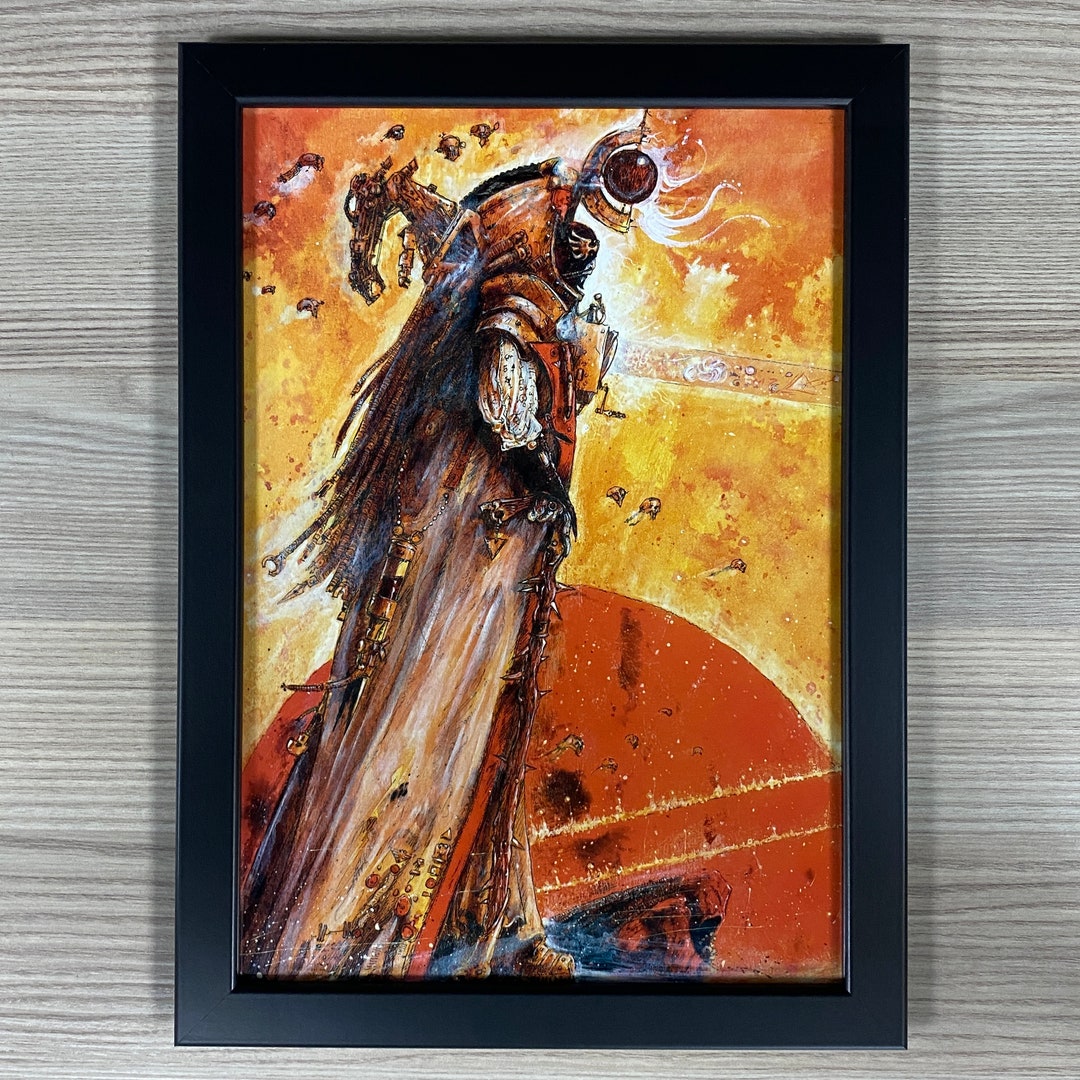The image is a detailed painting centered on a light gray wall. It features a tree-like figure with a brown, bark-less stump body suggestive of a person or being. The figure is adorned with an orangish helmet at its top, which resembles a space helmet, indicating a science fiction or futuristic theme. Flowing out from behind the helmet is hair alongside an orange extension that loops upward and back down. Below the helmet, on the chest, there is a yellowish component from which a line extends outwards and downward, resembling a limb. This figure's right arm descends in white, with a discernible hand. The scene is vibrant with colors where fiery orange, yellow, and white dominate the background, evoking a sense of flames or cosmic energy. There's a significant detail at the bottom with a rust-colored semicircle, potentially depicting a planet or sun, that arcs from the bottom left around the figure's waistline and culminates in a red dome shape. Above the helmet, a red ball, which could be a sun or planet, holds a line stretching to the edge of the painting, completing its abstract yet intricate composition.